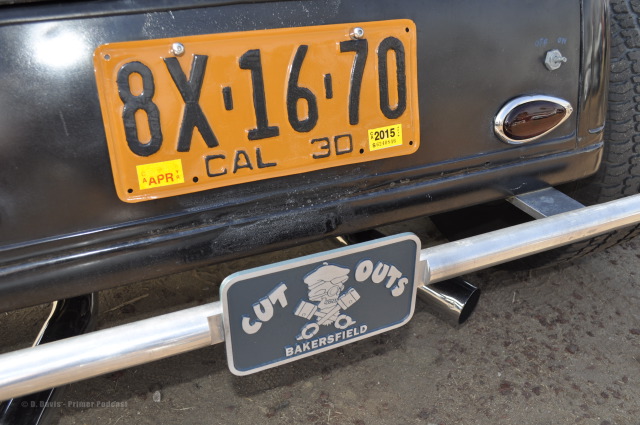This is a detailed color photograph of the back of a black or dark brown vehicle, possibly taken inside a garage during the daytime, with pavement visible underneath. The license plate is yellow and prominently displays the number 8X1670 with "CAL30" written below it. On the bottom left corner of the license plate, there's a yellow sticker with red text reading "APR," and on the bottom right corner, there is another yellow sticker with black text showing "2015." Beneath this main license plate, there is a smaller, black vanity plate bordered in silver, which reads "Cutouts Bakersfield." In the center of this vanity plate, there is an illustration of a skull and crossbones, with the skull turned to the right, wearing sunglasses, and sporting a painter's hat. The skull also appears to have a pair of handcuffs or boxing gloves. Additionally, there is an on-off switch positioned above a light on the back right side of the vehicle. The photo also captures one of the vehicle’s brake lights and a non-original muffler. There is a camera flash visible on the surface of the vehicle's rear.